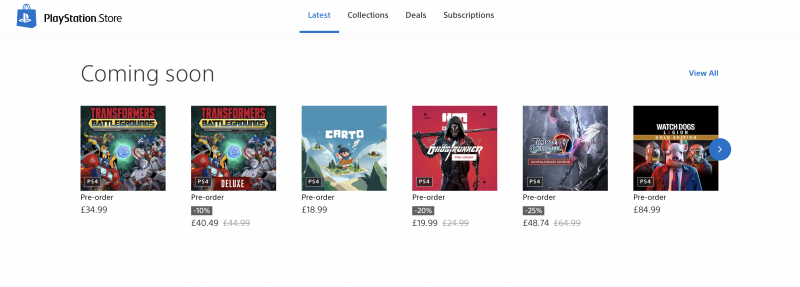A wide screenshot of the PlayStation Store is displayed, showcasing the "Latest" tab among other options like Collections, Deals, and Subscriptions. The store banner highlights six games under the "Coming Soon" section. The titles featured include "Transformers Battlegrounds" and its deluxe edition, "Carto" (in smaller text), a game resembling the name "Dead Runner" featuring an undead character with a stick slung over his shoulder, perhaps ready for combat, and a "Watch Dogs" game, noted to be a deluxe edition priced at £85. The final title appears to be too small to decipher but may be a fighting game or JRPG. Prices are listed in British Pounds, with some games on sale offering discounts of 10%, 20%, and 25%. All titles are for the PS4, reflecting a mix of new releases and premium editions.